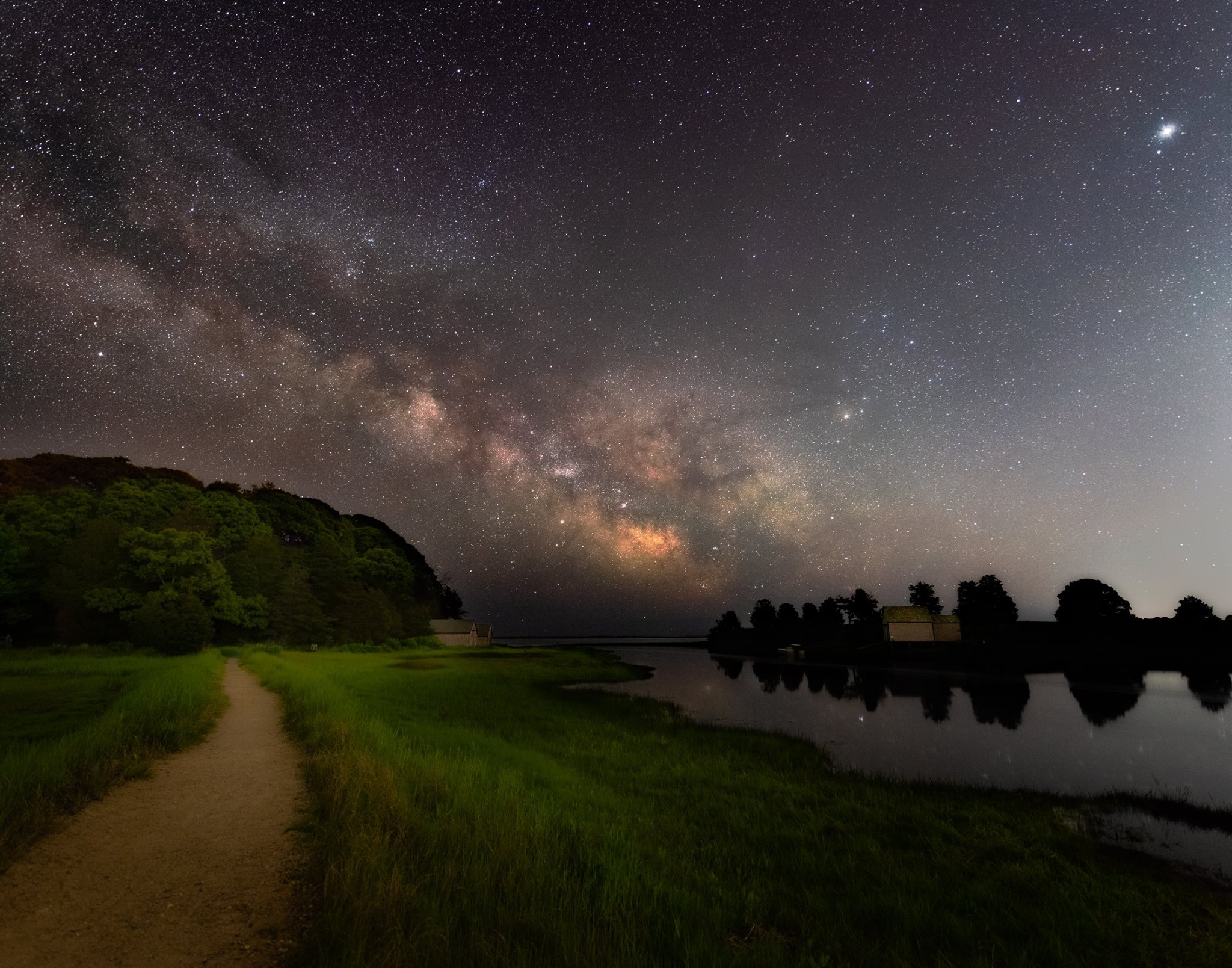The night sky, a vast expanse of black, is adorned with countless stars, painting a mesmerizing picture of the galaxy visible from this rural area. The celestial display features intricate orange hues of stardust scattered amongst the stars. On the left side of the image, a dirt path meanders into a densely wooded forest, while a building stands quietly in the distance. The right side is bordered by a tree line, framing the landscape. A body of water mirrors the ethereal sky, enhancing the tranquility of the scene. This photo captures the serene beauty of the nighttime countryside, where the vastness of the universe meets the quiet stillness of nature.